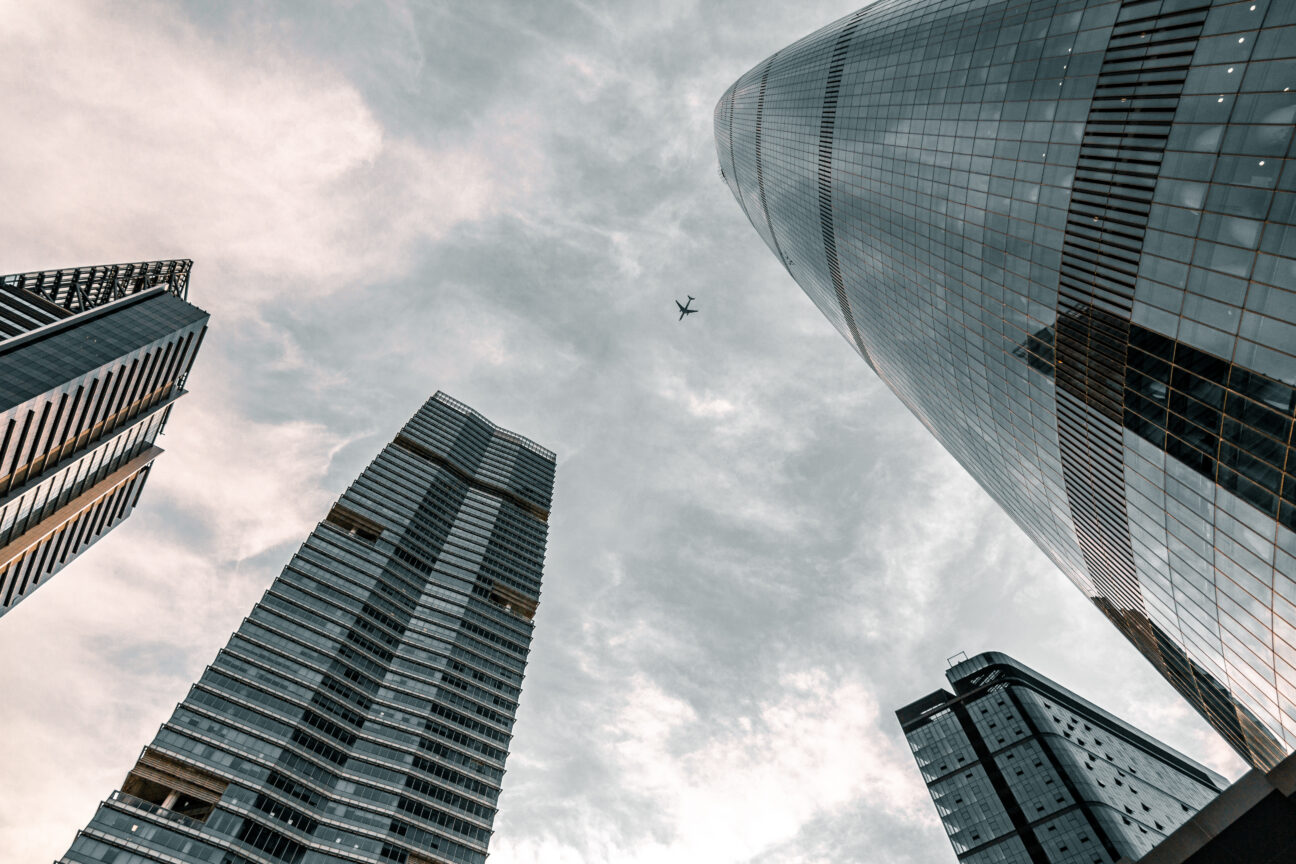The photograph captures an urban scene from the unique perspective of looking upwards from the ground. Dominating the image are four towering skyscrapers, each varying in height and style. The tallest building, with a sleek glass facade, protrudes dramatically from the right side of the frame. Another skyscraper, slightly set back in the background, has numerous floors, characterized by its commercial appearance of metal and mirrored windows. On the left, two more buildings stand prominently; one has visible balconies, suggesting residential apartments, while the other, slightly smaller, also features balconies extending from its facade.

The sky above is a patchwork of gray and white clouds, dense enough to obscure a clear view of the sky, yet brightened by sunlight diffusing through. Crowning the scene at the very top of the image, a jet airplane soars silently, its silhouette dark against the cloudy backdrop, adding a dynamic element to the otherwise static cityscape.